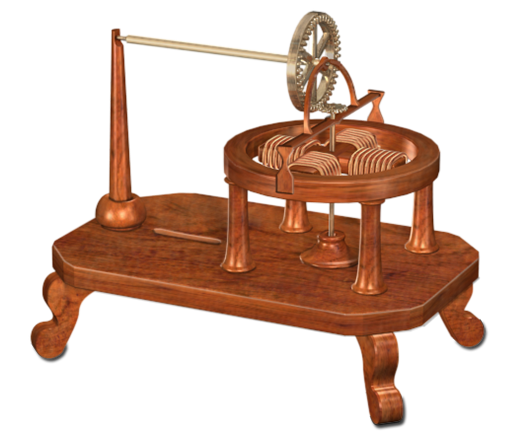This image depicts a detailed digital illustration or drawing of a vintage device, possibly resembling an old-time sewing machine or an early electric motor, set against a completely white background. The device is perched on a small table-like structure with short, curved, wood-colored legs, though the material could be copper, giving it a metallic sheen.

At the top of this structure, there's a small circular platform supported by wood-colored legs. Prominently featured is a curved, horizontal metal piece in a bronzy silver color, extending to connect with a metal gear. This gear, also in a silvery hue, plays a central role in the mechanism.

Additional details include a diagonal arrangement of copper wires, creating a cross-pattern effect. These wires seem to be part of the device's intricate assembly. At the base of the prominent gear, a horizontal metal stick connects it to another component, suggesting a link between various mechanical parts.

Overall, the image captures the complexity and vintage aesthetic of this mechanical device, highlighting its curious blend of wood-like and metallic elements, all carefully illustrated to offer a detailed and intriguing view.